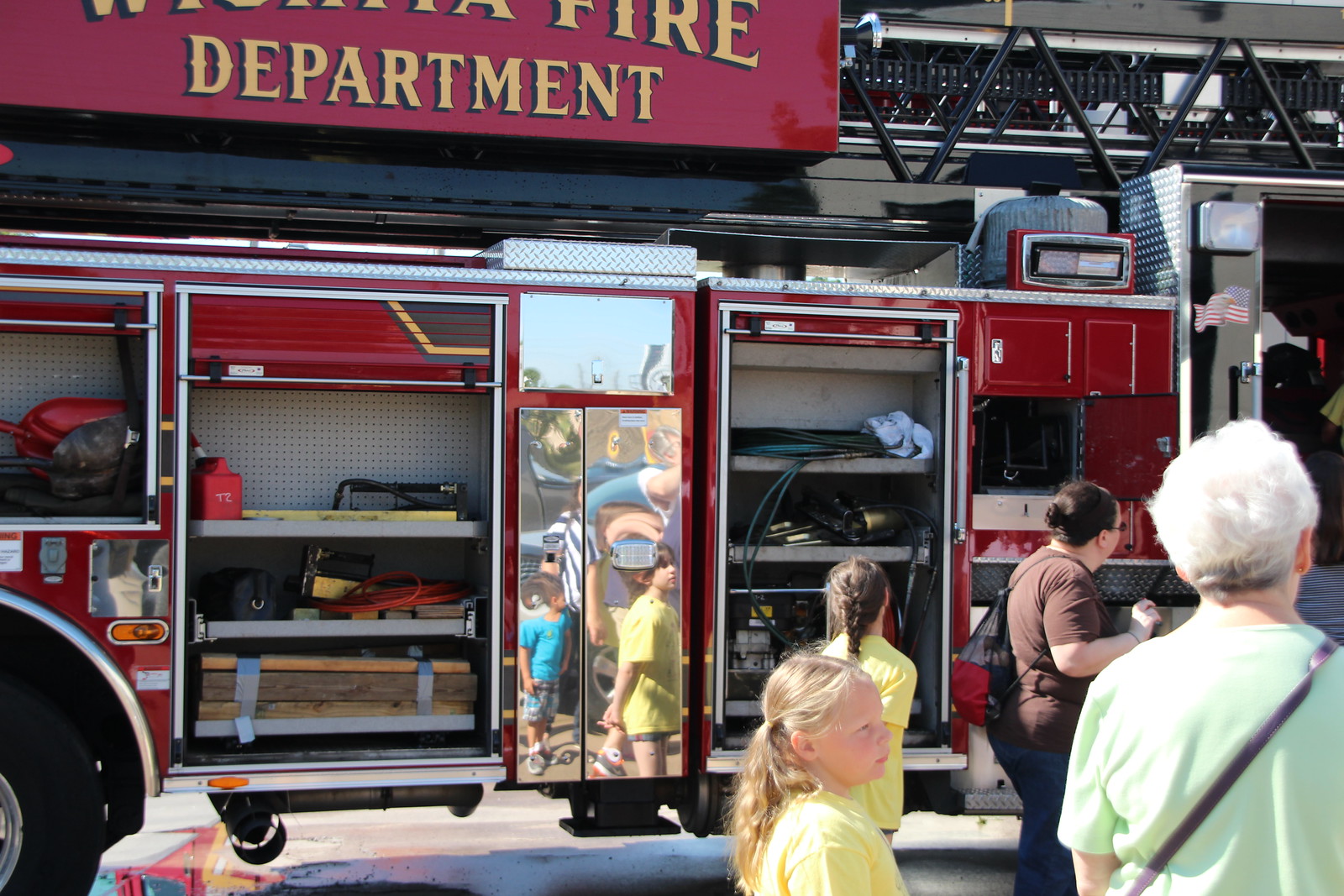The colored photo depicts a side view of a fire truck with its red and chrome compartments opened, showcasing various firefighting tools such as wood, gasoline containers, shovels, power tools, hoses, and ropes. The truck, which has railings atop and a partially visible red sign reading "fire department" in yellow block text with a black outline, features a mirrored door that reflects the scene. In front of the truck, several people are intently inspecting the compartments. Prominently, two young girls in yellow t-shirts stand beside an older woman with gray hair, who has a strap, likely from a purse, over her shoulder. A woman wearing a dark shirt, dark pants, and a string backpack with her hair up in a bun is also present. The scene suggests an event at the fire department, with both children and adults attending and engaging with the display.